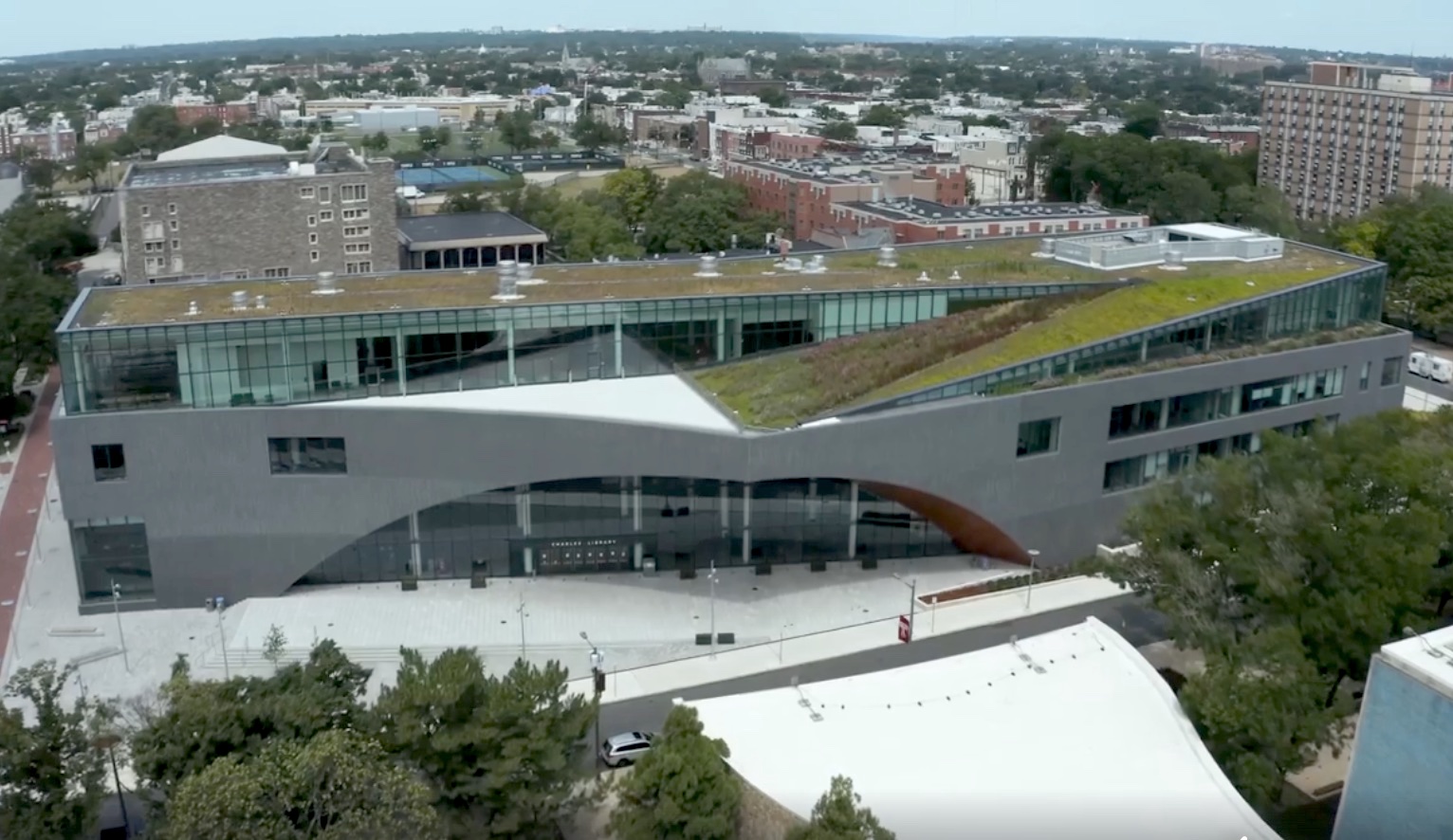This is a detailed aerial photo, likely taken from a neighboring tall building, overlooking an urban landscape during the daytime. The centerpiece is a distinctive graystone building with a unique architectural design. The structure is rectangular with a flat and slanted roof, featuring an elongated, semi-circular front entryway lined with multiple glass windows. The building's facade showcases additional arched concrete detailing, and below, there is a long rectangular entry area filled with doors.

The flat roof has been transformed into an urban garden, with lush green grass planted on both the flat and slanted portions. This garden is framed by metal pipes, and a fenced-off air conditioning center is visible. A notable diagonal ramp extends from the center to the right-hand side of the roof.

Surrounding this building, the cityscape includes numerous apartment buildings and roads. On ground level, a mixture of white concrete, gray asphalt roads, and a red sidewalk are visible, as well as clusters of trees, giving the scene a touch of greenery against the urban backdrop. The blue sky above completes the vibrant city view.